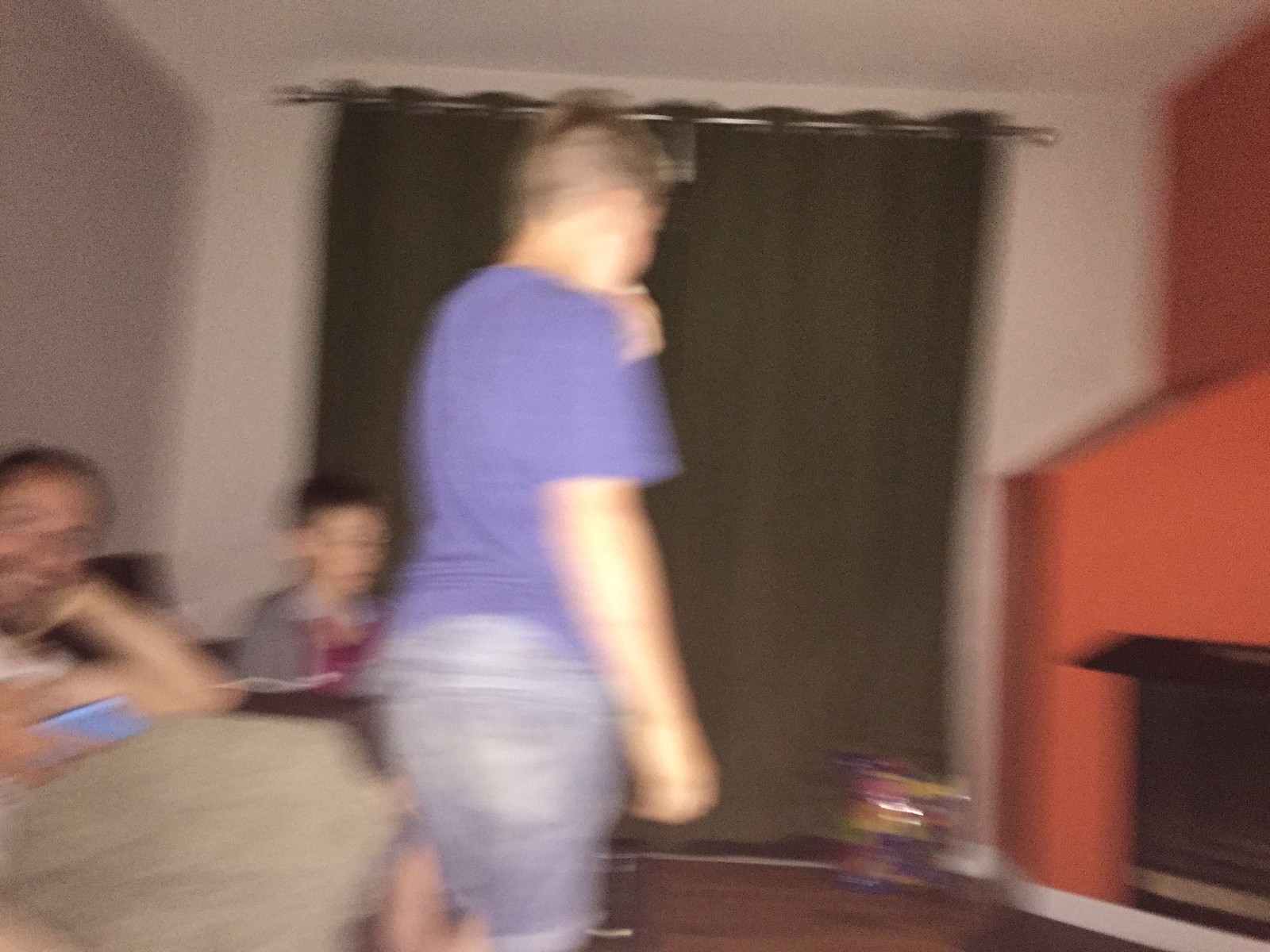This is a blurry photograph of a living room, likely from the late 1950s or early 1960s. On the right side of the image, there's a prominent fireplace bordered by an angled, bright red structure emerging from the wall. The back wall features a large window dressed in dark brown curtains hanging from a wooden rod, set against a tan wall. The left side of the room, with its white walls, hosts a black couch.

There are three people in the image. In the center foreground stands a boy (or possibly a young girl) with short hair, wearing a blue t-shirt and denim shorts, their back turned towards the camera. To the left, sitting on the couch, is a younger boy with dark hair, wearing a gray shirt with a hint of red in the center. Next to him is a man with a mustache, beard, and possibly glasses. The man has a tan object, perhaps a pillow or blanket, on his lap, and he's holding a phone in his right hand while his left hand supports his chin. He is smiling directly at the camera.